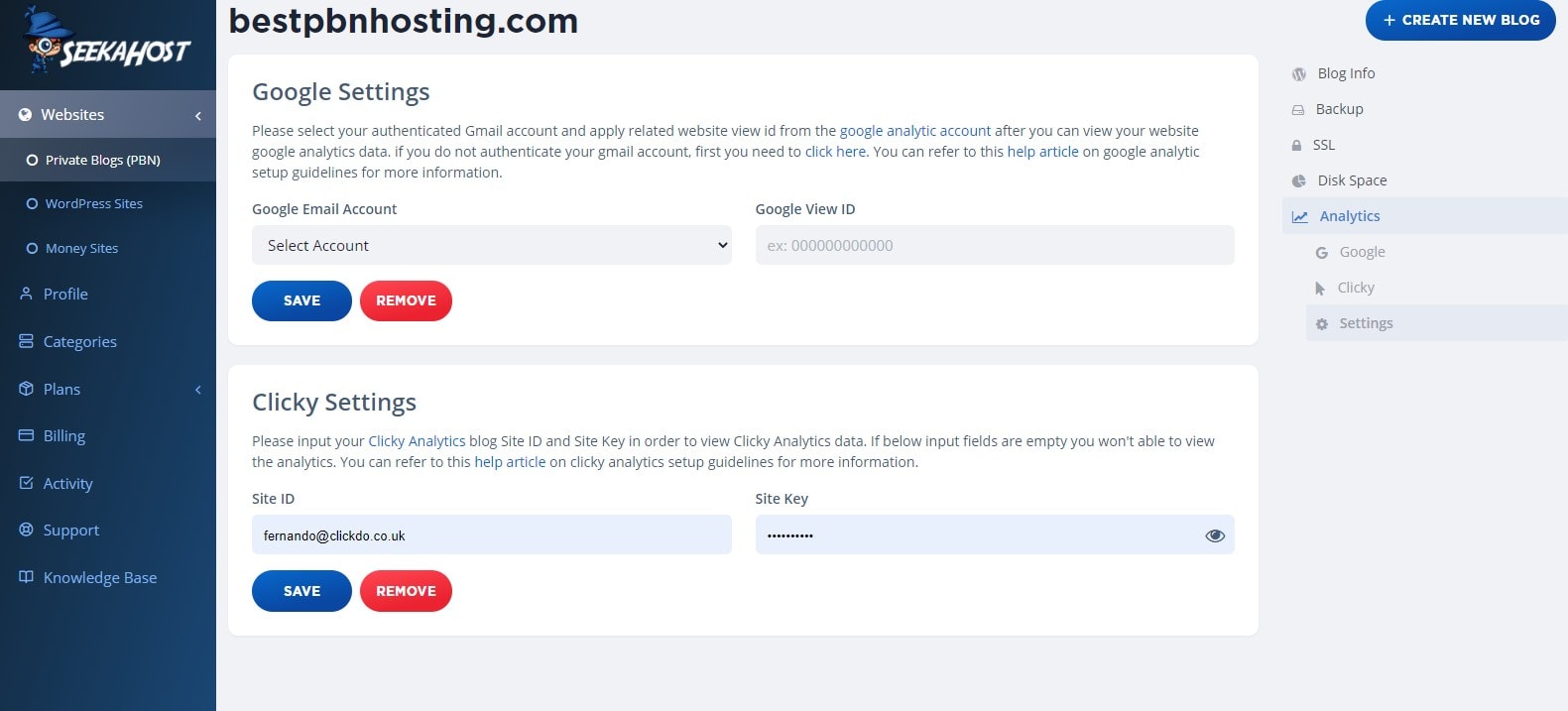This image showcases a detailed view of the Sika Host website interface. In the upper left corner, the Sika Host logo prominently appears—a figure donned in a blue costume and hat, holding a magnifying glass, with "Sika Host" written in white text beside it. The background of the page is primarily blue, giving it a cohesive and professional appearance.

At the top of the page, the URL "bestpbnhosting.com" is displayed, indicating the specific hosting service being presented. On the far right side, a vibrant red button invites users to "Create New Blog."

The left-hand column features a range of navigational options in white text: "Websites," "Private Blogs," "PBN," "WordPress Sites," "Money Sites," followed by categories for "Profile," "Categories," "Plans," "Billing," "Activity," "Support," and "Knowledge Base." 

In the center of the page, under "Google Settings," users are prompted to authenticate their Google account to access and manage their Google Analytics data. A step-by-step instruction reads: "Please select your authenticated Google account and apply the related website view ID from the Google Analytics account. After authentication, you can view your website's Google Analytics data. If you do not authenticate your Gmail account, first you need to click here," with "click here" highlighted in blue for easy access to the help article on Google Analytics setup guidelines.

Below this, there's a section designated for selecting a "Google Account" from a dropdown, accompanied by blue "Save" and "Remove" buttons. Another section beneath this, titled "Clicky Settings," elaborates on setting up Clicky Analytics, similarly offering a blue "Save" button and a red "Remove" button for managing the settings.